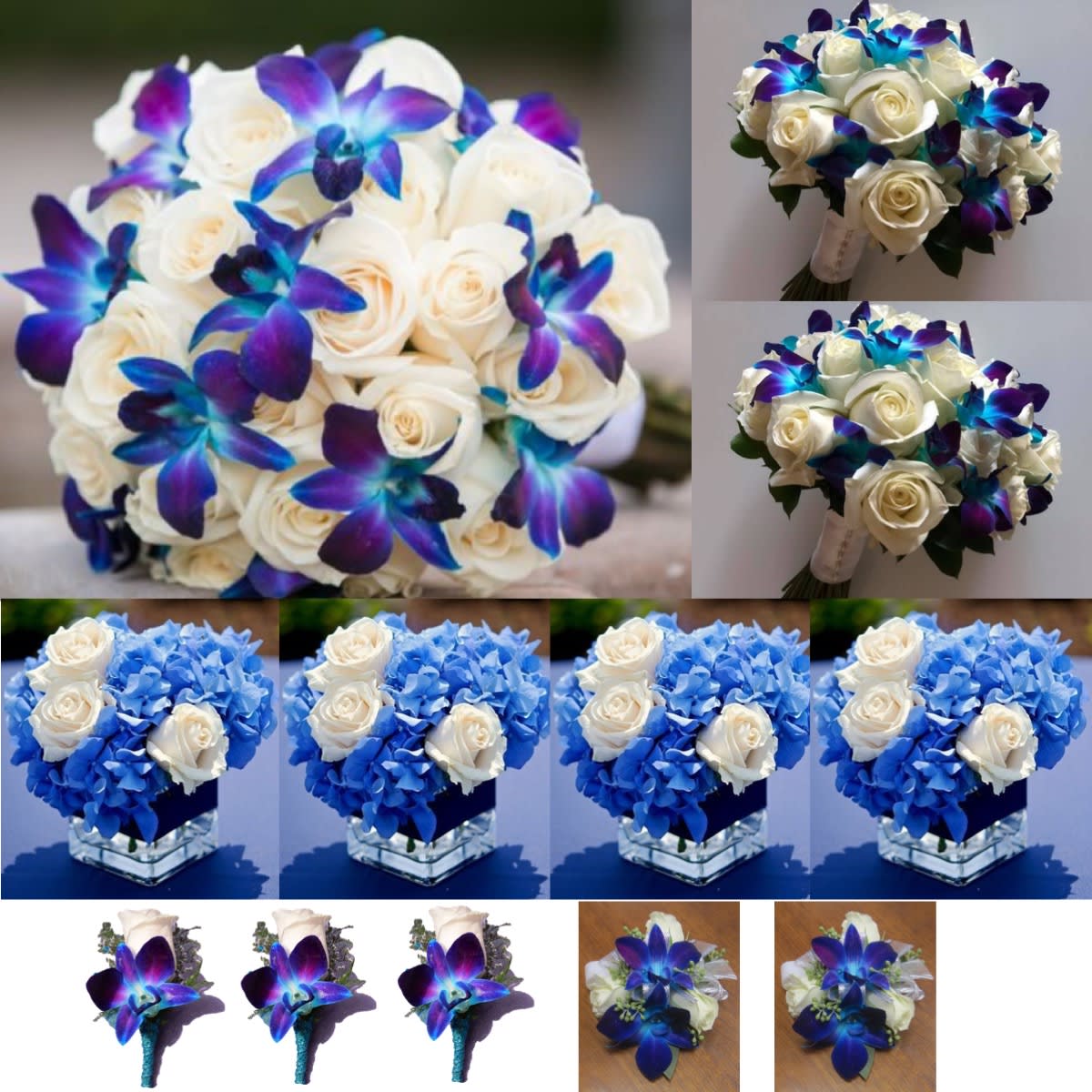The images collectively depict an array of exquisitely arranged wedding bouquets and decorative flower arrangements. Central to the composition is a large photo at the top left, showcasing a bouquet dominated by white roses interspersed with vibrant purplish-blue flowers, which appear almost luminescent as they contrast with the natural tones of the roses. To the right of this main image are two smaller photos capturing different angles of the same bouquet, highlighting its intricate details. Below these, a row of four photos displays a consistent tabletop arrangement featuring white roses nestled among turquoise-blue flowers in a glass, square vase. At the bottom, there are two detailed shots of brooches and three single flowers to the left, all cohesively embodying similar color themes of white, blues, and purples. These elements, indicative of a special and elegant event such as a wedding, are meticulously positioned to emphasize their aesthetic appeal and harmony.